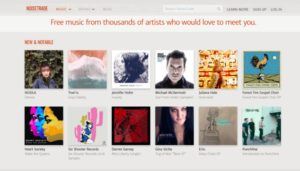Here's a descriptive caption based on the voice-described image:

"This is a screenshot of a website's header and main content area. The top of the page features a grey background with a navigation bar. On the left side of this navigation bar, there is an orange logo. To the right of the logo, there is an orange hyperlink followed by two grey hyperlinks. On the right side of the navigation bar, there is a white search bar, flanked by three grey hyperlinks. Below the navigation bar, a white horizontal section spans the width of the page, containing the message, 'This is free music from thousands of artists who would love to meet you.' Beneath this, there is a section title in orange font, followed by a grid of thumbnail images arranged in two rows of six."